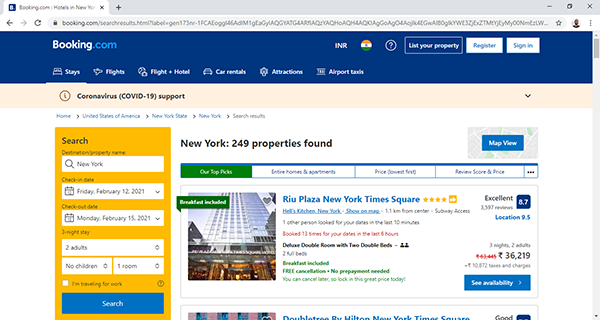The image depicts a browser with a single open tab showing the Booking.com website. The tab's title reads "Booking.com - Hotels in New York." The website's top blue navigation bar prominently displays the Booking.com logo on the left, with options on the right including currency selection marked as INR (Indian Rupee), a help icon indicated by a circle with a question mark, and buttons labeled "List your property," "Register," and "Sign in." Below this is a brown horizontal banner highlighting "Coronavirus (COVID-19) support" on the left side.

The main content area features a section with a white background where users can conduct their search. Fields include "Destination: New York," "Check-in: Friday, February 12th, 2021," "Check-out: Monday, February 15th, 2021," "Two adults," "No children," "One room." These fields are outlined in yellow, with a blue "Search" button located at the bottom.

On the right side of the content area, the site displays information that New York has "249 properties found." The property listing categories include "Our top picks," "Entire homes and apartments," "Price (lowest first)," and "Review score and price." The only visible property in the image is "Riu Plaza New York Times Square," rated with four stars. Additional details about this property mention its location in Hell's Kitchen, New York, its proximity being 1.1 kilometers from the city center, and access to the subway.